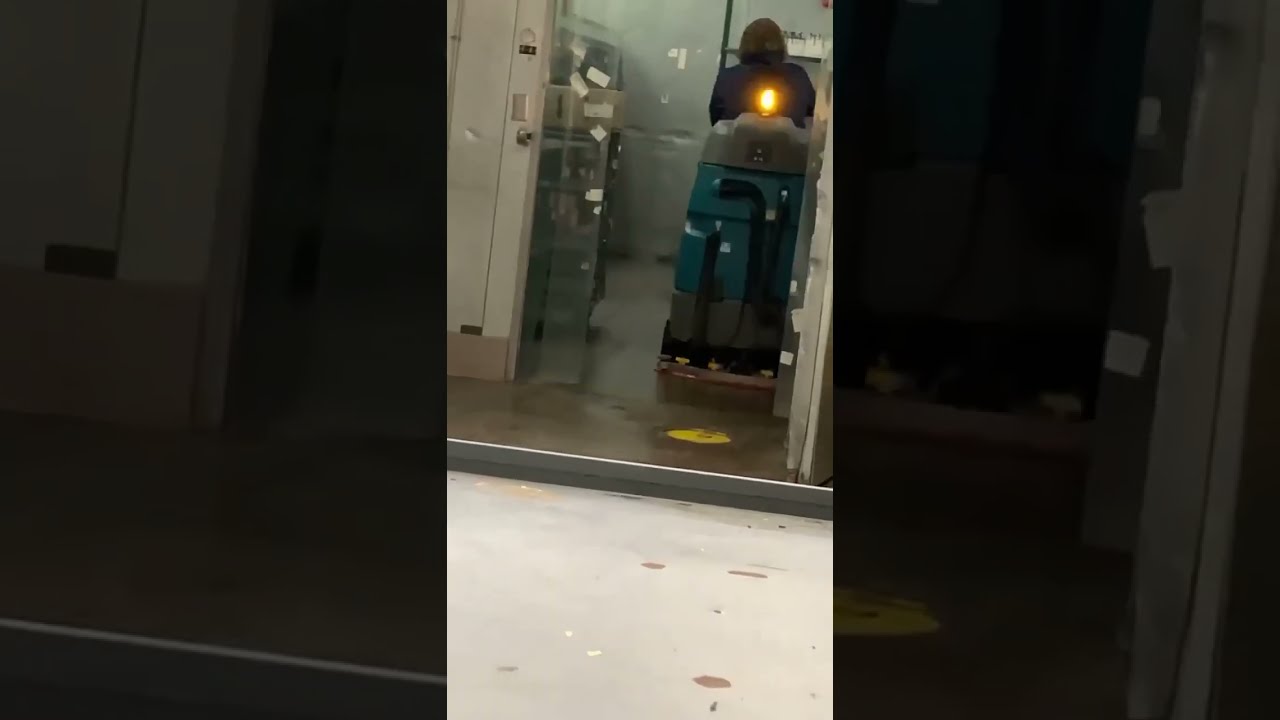The image depicts an indoor area where a custodian is operating a large floor cleaning machine. The machine, a mix of dark blue, turquoise, and gray, prominently features hoses and a light at the top, which is illuminated, suggesting that the cleaning is actively taking place. The scene captures the reflection of the machine in a distant glass door, adding depth to the composition, while several pieces of colored paper (green, purple, brown, off-white, black, gray, yellow, tan) are stuck to the glass. The background includes a metallic door or wall, suggesting an industrial or commercial setting. The floor transitions from a light gray with brown spots to a darker brown, separated by a gray-bordered step. The layout of the photograph includes a central image flanked by close-up segments, creating a wide rectangular presentation. The overall tone of the image is casual, as it lacks professional polish and any textual information.